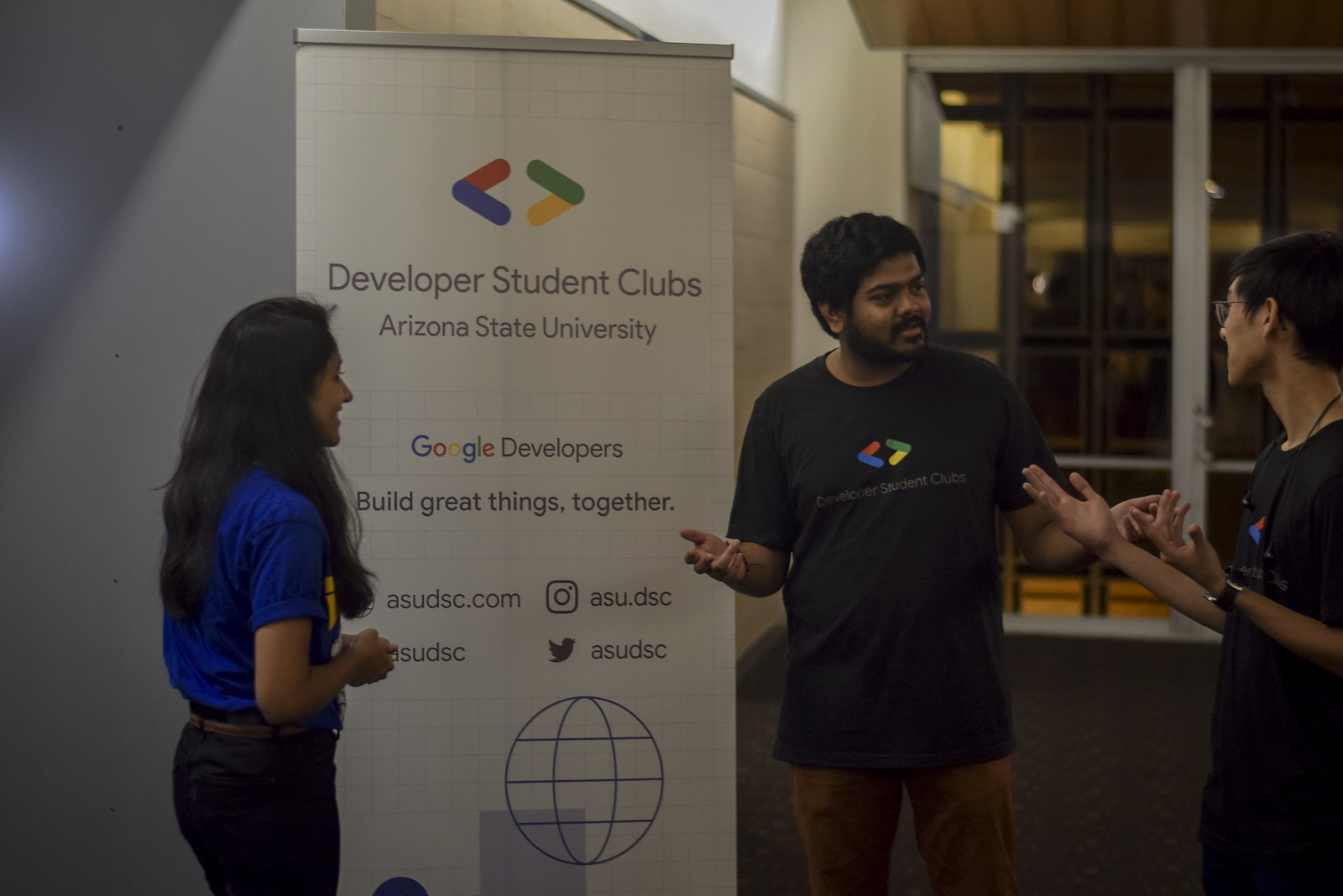The image depicts a student event taking place at night in a well-lit indoor corridor, possibly an auditorium or office, with a white and gray wall and a large glass door in the background. In the foreground stands a vertical banner adorned with the logo of greater-than and less-than signs in Google’s colors: red, blue, green, and yellow. The banner's headline reads "Developer Student Clubs" with a subheading "Arizona State University," followed by "Google Developers," "Build great things together," and the website "asudsc.com." Below this are the Instagram and Twitter handles "@asu.dsc" and a globe design with lines and patterns.

Three individuals are gathered around this banner. On the left, a young Indian woman with long black hair, wearing a blue t-shirt and black pants, smiles at the others. At the center, an Indian man with black hair and a beard, clad in a black t-shirt displaying the same logo and text as the banner, brown trousers, and black socks, engages in animated conversation. To his right, another man, clean-shaven with short black hair and glasses, wears an identical black t-shirt and has earphones around his neck, along with a wristwatch. This man mirrors the animated gestures of the first, contributing to the lively interaction. The cohesive appearance of the black t-shirts, each adorned with the emblem and relevant text, underscores the united theme of the Developer Student Clubs event at Arizona State University, supported by Google Developers.